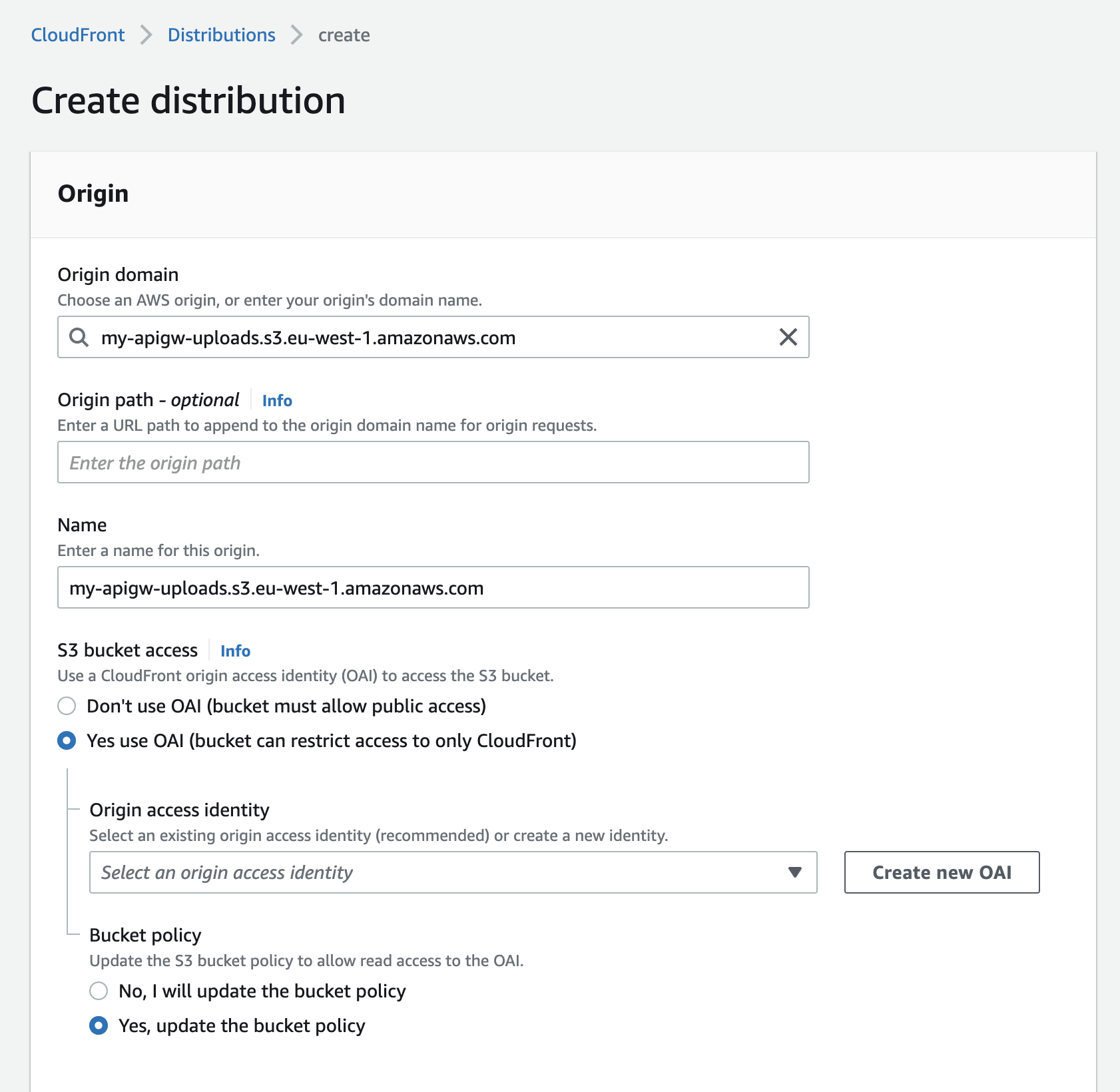### Detailed Caption for Screenshot

The image is a detailed screenshot from an app or program interface for creating a distribution in AWS CloudFront.

**Background and Header:**
- The background is predominantly light gray.
- At the top left, there are breadcrumb links:
  - "CloudFront" in blue
  - Followed by a gray greater-than symbol (`>`)
  - "Distributions" in blue
  - Another gray greater-than symbol (`>`)
  - "Create" in dark gray and lowercase

**Main Heading:**
- Prominently in bold black letters, the title "Create Distribution" is displayed just below the breadcrumbs.

**First Subsection - Origin:**
- Enclosed in a white background with a light gray border at the top, the subsection is titled "Origin" in smaller bold black letters.
  - Below this, there is a gray line separating the title from the content.

**Origin Domain:**
- The field is labeled "Origin Domain" in standard black paragraph text.
- Below the label is instruction text in smaller, lighter gray: "Choose an AWS origin or enter your origin's domain name."
- Within a black-outlined rectangle with a white background:
  - The user has entered "my-apigw-uploads.s3.eu-west-1.amazonaws.com".
  - To the left, there's a search icon.
  - To the right, there's an X icon for clearing the input.

**Origin Path - Optional:**
- To the right of the label is an "Info" link in blue.
- Below, there's smaller gray instructional text: "Enter a URL path to append to the origin domain name for origin requests."
- A text field with a gray outline prompts with placeholder text "Enter the origin path."

**Name:**
- Labeled "Name," with instructional text prompting to enter a name for the origin.
- Similar to the Origin Domain field, it is outlined in black with the same example input.

**S3 Bucket Access:**
- Labeled in bold "S3 Bucket Access" with an "Info" link in blue.
- Below is an instruction in small gray text: "Use a CloudFront origin access identity (OAI) to access the S3 bucket."
- Two radio buttons:
  - The first option (not checked): "Don't use OAI (bucket must allow public access)."
  - The second option (checked): "Yes, use OAI (bucket can restrict access to only CloudFront)."

**Origin Access Identity:**
- Labeled in black followed by a dark gray subtext.
- A dropdown menu inside a rectangle with the text "Select an Origin Access Identity."
  - To the right of this menu, a button labeled "Create New OAI."

**Bucket Policy:**
- Further subtext provides additional guidance.
- Two radio buttons:
  - The user has selected the second option: "Yes, update the bucket policy."

The meticulous detail in this caption aims to provide clarity on each element visible in the user's interface.